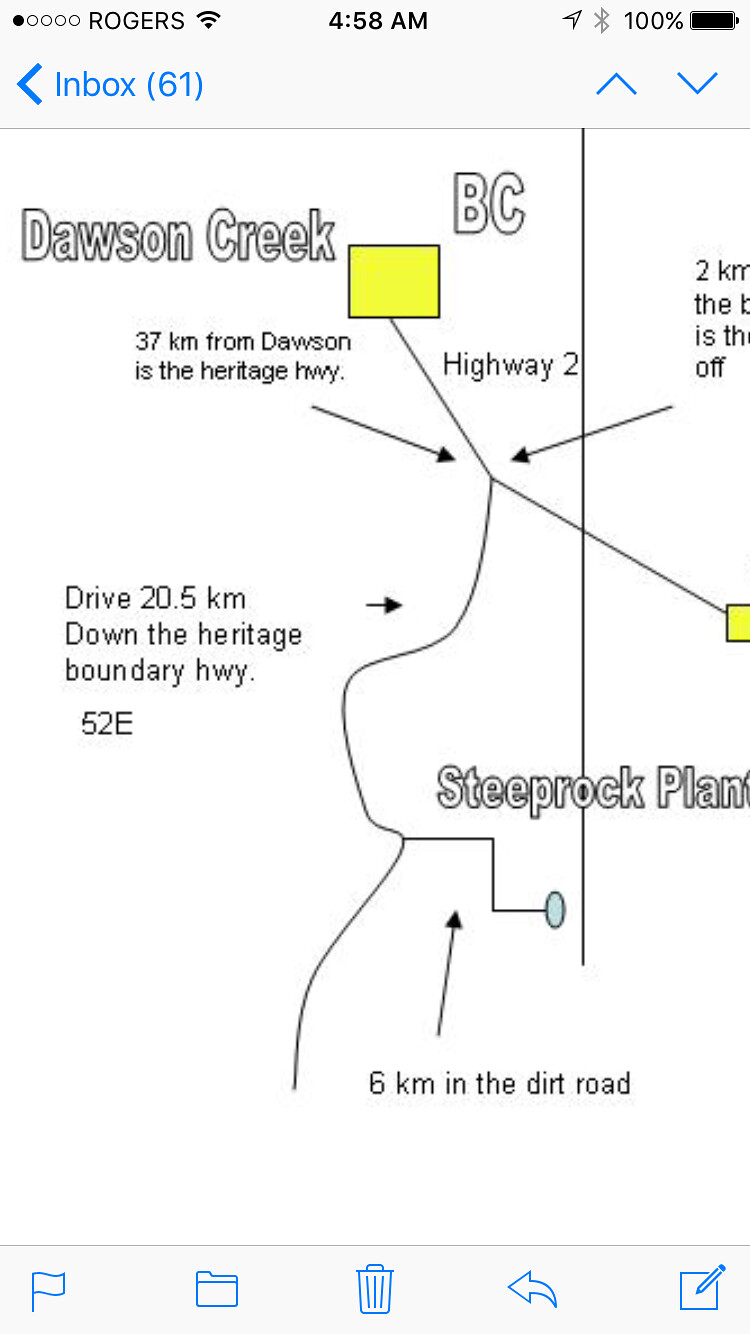This image is a screenshot taken from a cell phone, displaying various status indicators and content. At the top of the screen, it reads "Rogers," indicating the network provider, with one bar of signal strength, showing the time as 4:58 AM. The battery icon indicates a full 100% charge. Below this, there's a header stating "INBOX (61)" in blue text, suggesting there are 61 unread emails.

The primary element of the screenshot is a map that includes directional information. The map prominently features the text "Dawson Creek, BC," with an adjacent yellow box. Key navigation details include the instruction to travel "37 kilometers from Dawson to the Heritage Highway, Highway 2." Further directions specify driving "20.5 kilometers down the Heritage Boundary Highway 52 E," and continuing "6 kilometers on a dirt road." Other notable landmarks include "Steep Rock Plantation."

At the bottom of the screen, there are several clickable icons in blue: a flag, a folder, a trash bin, a share button, and a writing tool symbol.